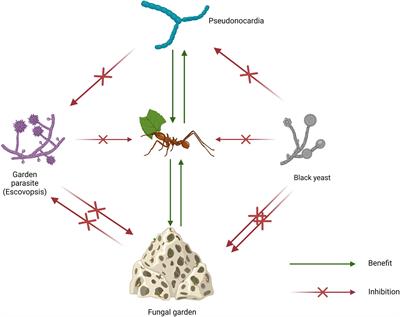The image is a detailed scientific diagram illustrating the interactions within an ant's ecological system. At the center of the image is an ant, which serves as the focal point. Surrounding the ant are various labeled images connected by arrows, indicating their ecological relationships. 

To the right of the ant is a depiction of gray stalks labeled "Black Yeast." Below the ant, there's a white, sponge-like structure labeled "Fungal Garden." To the left of the ant is an image of purple branches labeled "Garden Parasite." Above the ant, a blue-colored structure labeled "Pseudonocardia" is illustrated. The arrows connecting these images are color-coded: green for vertical connections and red for others. 

The diagram includes various textual annotations such as "pseudonocardia," "black yeast," "fungal garden," "garden parasite," "escovopsis," "benefit," and "inhibition," illustrating the complex interactions and processes occurring within this microscopic ecosystem. The colors used in the diagram are diverse, featuring red, green, brown, white, gray, purple, and bluish-green, and the setting suggests it is used for scientific purposes to explain the ecological relationships and processes involving the ant and its environment.